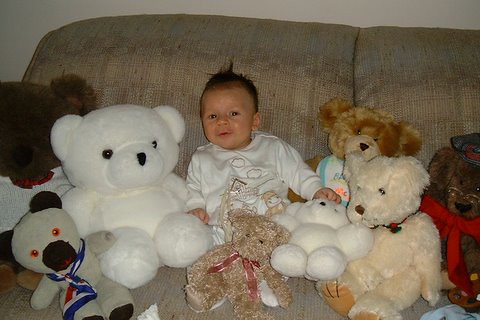In this charming amateur photograph, we see a baby, likely around one to two years old, sitting upright and smiling indoors on a light brown couch with a slight striped pattern and a high back. The baby's short dark hair is spiked upward, adding to the cuteness of the scene. The baby is clad in a white jumper adorned with little clouds and a small teddy bear illustration on the front. The background wall is beige or gray, making the scene feel warm and cozy.

Arrayed around the baby are numerous teddy bears of various sizes and colors. Immediately to the baby's left sits a large dark brown teddy bear wearing a white T-shirt. On the lower left, there's a brown and white teddy bear. Beside that, an older knitted white teddy bear with a brown face and ears, adorned with a red, white, and blue scarf. Next to it, a large white teddy bear with black eyes and a black nose cuddles close. To the right of the baby, we find a small white teddy bear, a medium-sized brown teddy bear wearing a bib, another light brown teddy bear, and a dark brown teddy bear. In the baby's lap rests a brown teddy bear with a red ribbon around its neck. 

The photograph is horizontally rectangular and softly illuminated by a flash, enhancing the indoor setting details. The absence of a date or other text suggests the timeless warmth of this candid, familial moment.